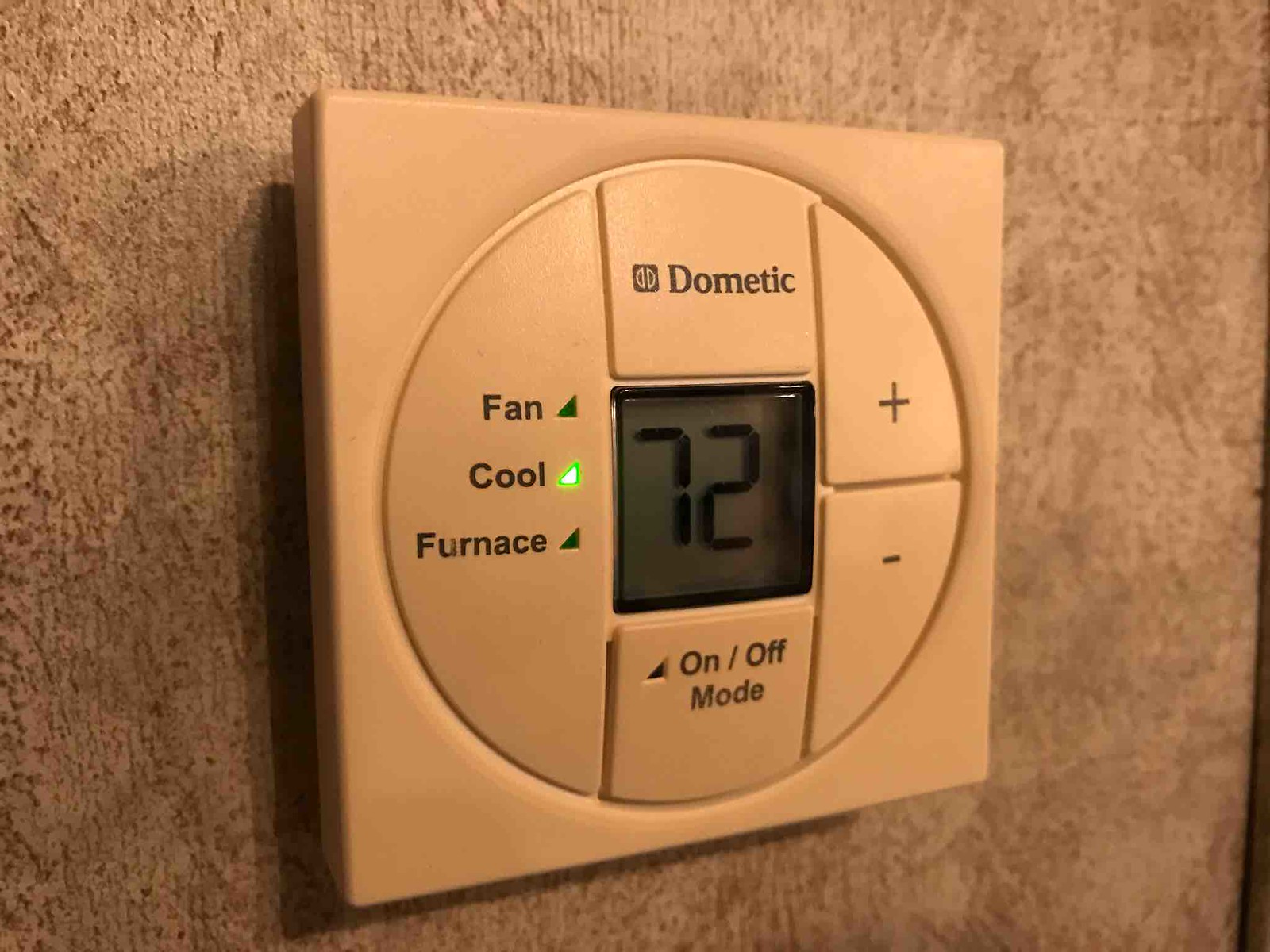This close-up photograph captures a Dometic thermostat, prominently displayed against a weathered wall. The wall itself is marked with several poke holes and etchings, suggesting age and a rough texture, possibly of old concrete or distressed wood. 

The thermostat features a square frame that encompasses a central circular control panel. Within this circular section, essential controls are laid out. To the left, there are labeled indicators for "Fan," "Cool," and "Furnace," with the "Cool" setting illuminated by a green light, signifying that the air conditioner is active. At the center of the display, a digital readout shows the current temperature, set to 72 degrees Fahrenheit.

Below the main display, there's an "On/Off" mode button, unlit in this image. Adjacent to the circular control panel on the right side, there are tactile buttons marked with a plus (+) and minus (-), allowing adjustment of the temperature setting. 

In summary, the image details a Dometic thermostat, characterized by its square structure and integrated circular control interface, set against a distinctly textured, aged wall.